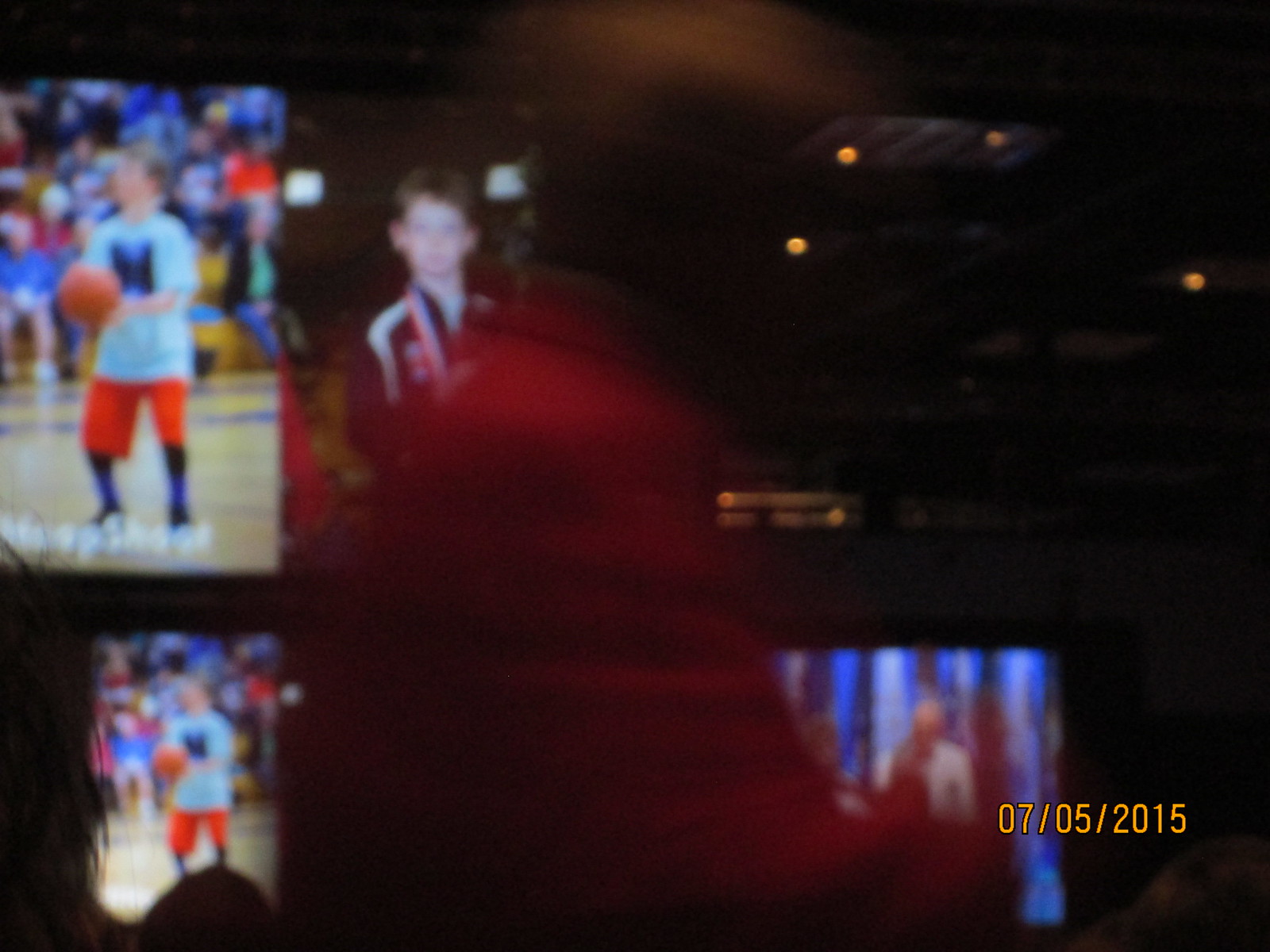On July 5th, 2015, the image captures a man in a red shirt walking past a series of out-of-focus and blurred screens displaying various photographs. These screens prominently feature a young boy dressed in orange shorts and blue socks, playing basketball. In one image, the boy is poised to take a shot, wearing a white shirt with a big blue "N." Another image shows a close-up of the boy's face, wearing a sash or possibly a medal over a track jacket. Below these, another screen repeats the shot of the boy about to take his basketball shot. There's also a screen on the bottom right displaying a person against a blue and white background. The entire scene appears to be part of a celebratory ceremony, rather than a somber event, perhaps commemorating the boy's achievements in basketball.